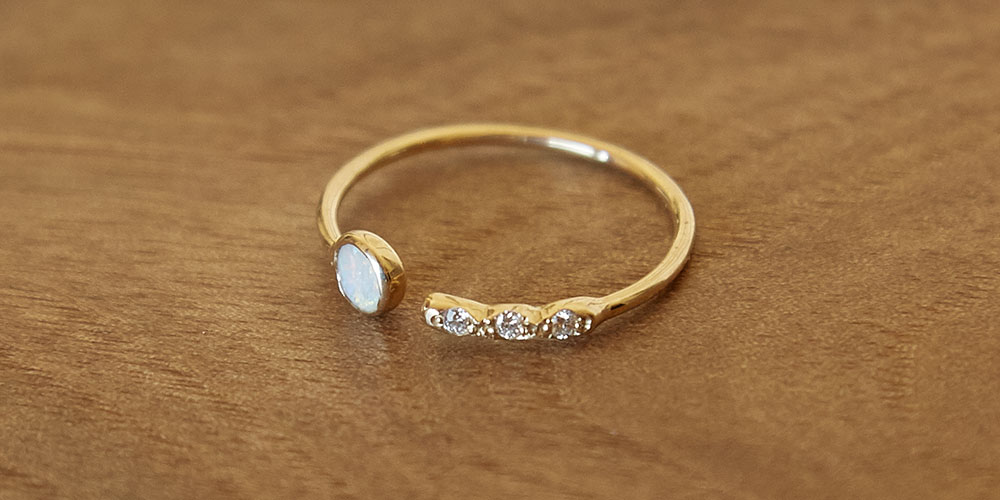The image depicts a close-up of a ring placed on a medium brown wooden table. The ring is crafted from what appears to be 14 karat gold, and it features an unusual design, being incomplete and open-ended. One end of the ring holds a prominent bluish gemstone, possibly resembling a diamond with a mother-of-pearl-like quality, which is flat and round in appearance. On the opposite end, the ring showcases three smaller, clear round diamonds set within the gold. The ring is rather skinny and delicate in structure, seemingly pliable due to its open design, with a small gap between the two ends. Additionally, there is a section inside the ring with a silver-colored detail, contrasting subtly with the predominant gold. The overall design suggests it is more of a cocktail ring than an engagement or wedding ring, emphasizing its unique and fashionable appeal.